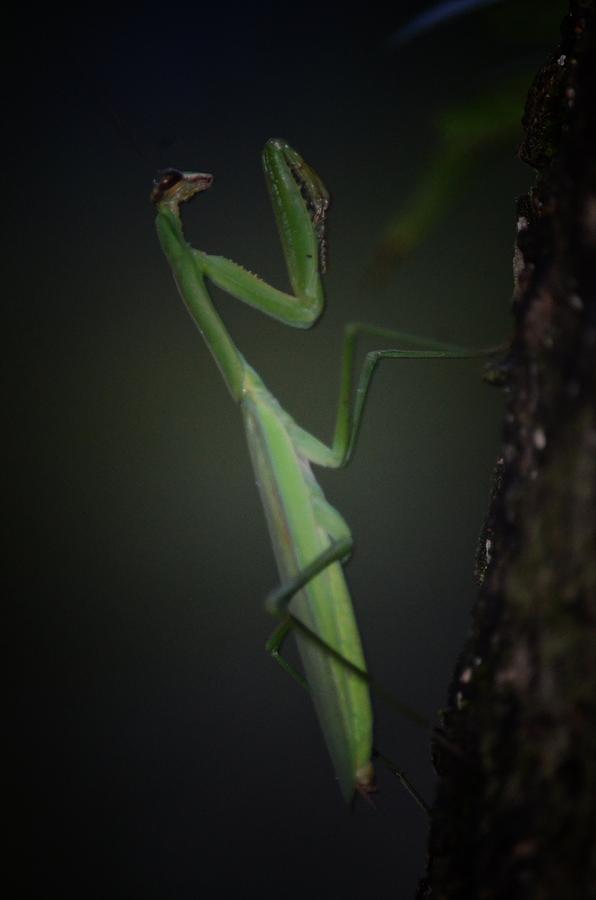This photograph captures an adult praying mantis climbing a textured tree or log. The image is quite dark and dim, suggesting it was taken at night, as details are challenging to discern. However, the mantis's defining features are visible: its signature claws, used for capturing prey, and its intricate legs equipped with thorns and hooks for holding its meal in place. The mantis exhibits a blend of green shades with a dark green tip, light green middle accented with white, and a green head displaying distinctive beady eyes. The background appears blurred and faded, primarily composed of muted greys and blacks, adding to the photo's overall dim ambiance. Despite the poor focus, the tree's bark is textured with shades of brown, black, and some white specks, adding to the natural setting of this nocturnal scene.